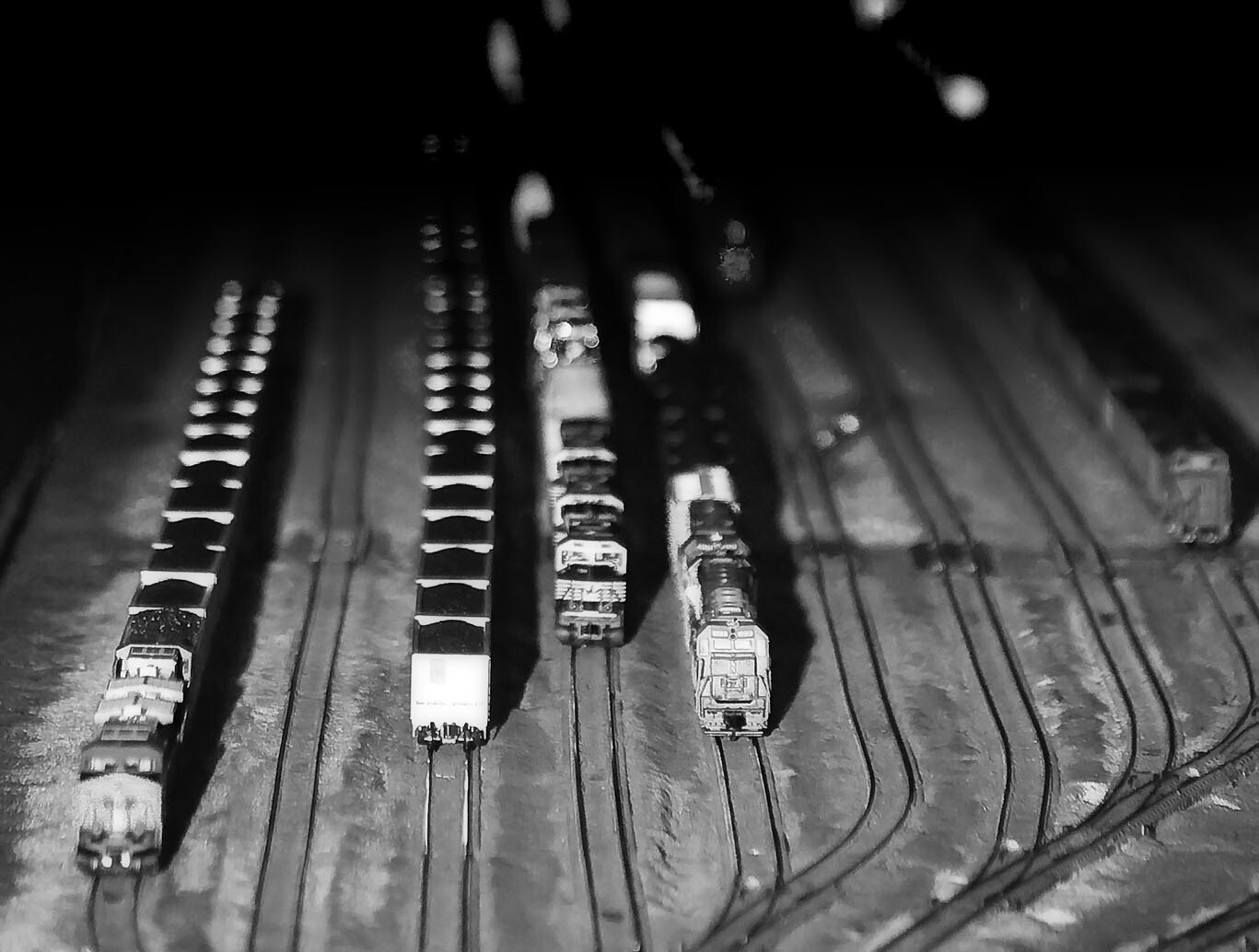The black and white photograph captures an aerial view of a model railroad, characterized by an intricate network of intersecting and curving miniature train tracks. The image's focus transitions from a clear, bright foreground to a dark, blurry background. The landscape features nine parallel tracks, several of which merge or curve towards the left. On these tracks, various toy trains are stationed: one on the far leftmost track (track one), three in the middle tracks (tracks four, five, and six), and another one on the far right (track nine). These miniature trains predominantly feature open-top cars, appearing to carry coal or gravel. The crisp detail in the foreground contrasts sharply with the obscured and shadowy back of the image, creating a sense of depth and scale within this meticulously arranged miniature train yard.